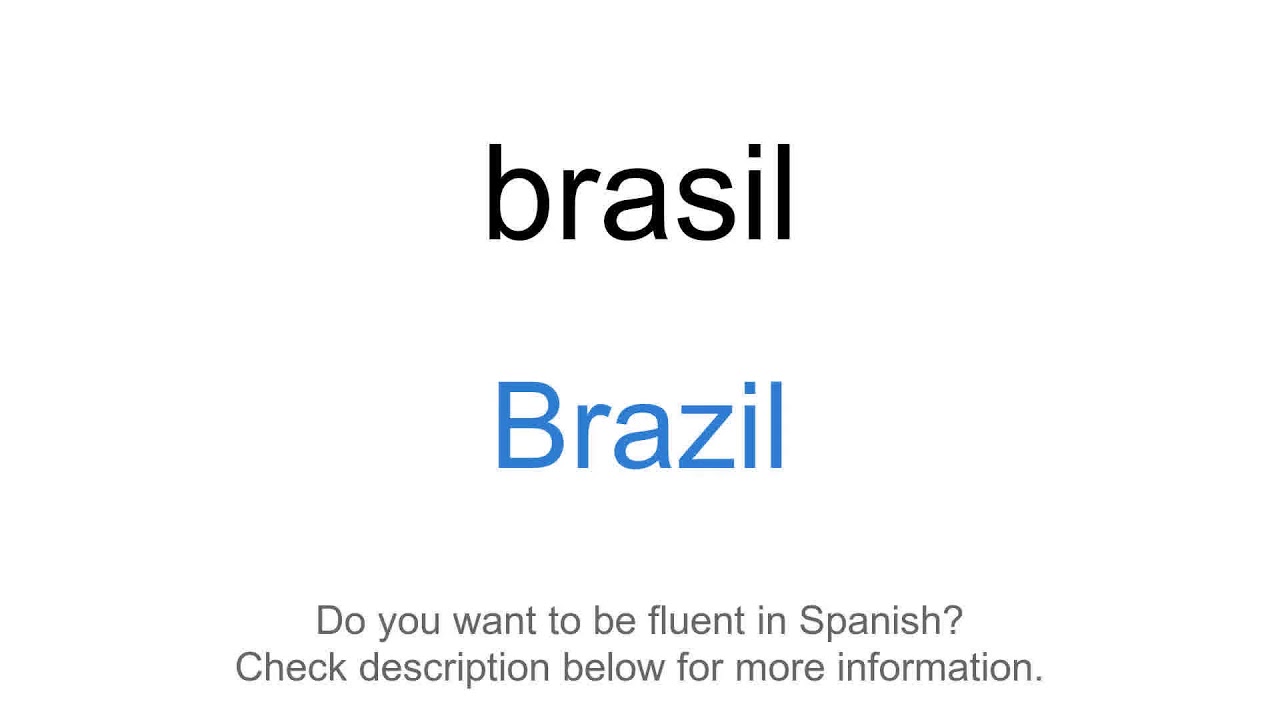The page presents a straightforward design with centered text. At the top, in a large black font, the word "brazil" is displayed in all lowercase letters. A few lines down, "Brazil" is written again, this time with an uppercase 'B' followed by lowercase 'r-a-z-i-l,' in a vibrant blue color. Both instances of the word "Brazil" share the same font size but differ in color and capitalization.

Further down the page, a smaller gray font poses the question, "Do you want to be fluent in Spanish?" On the following line, also in gray and the same smaller font, it says, "Check the description below for more information." These lines of text are also centered, aligning with the previously mentioned instances of "Brazil." However, the smaller text appears to be slightly left-aligned relative to the centered "Brazil" text, offering a subtle visual distinction.

Overall, this minimalist layout emphasizes the word "Brazil" prominently at the top, creating an engaging visual hierarchy that draws the viewer's attention sequentially down the page.